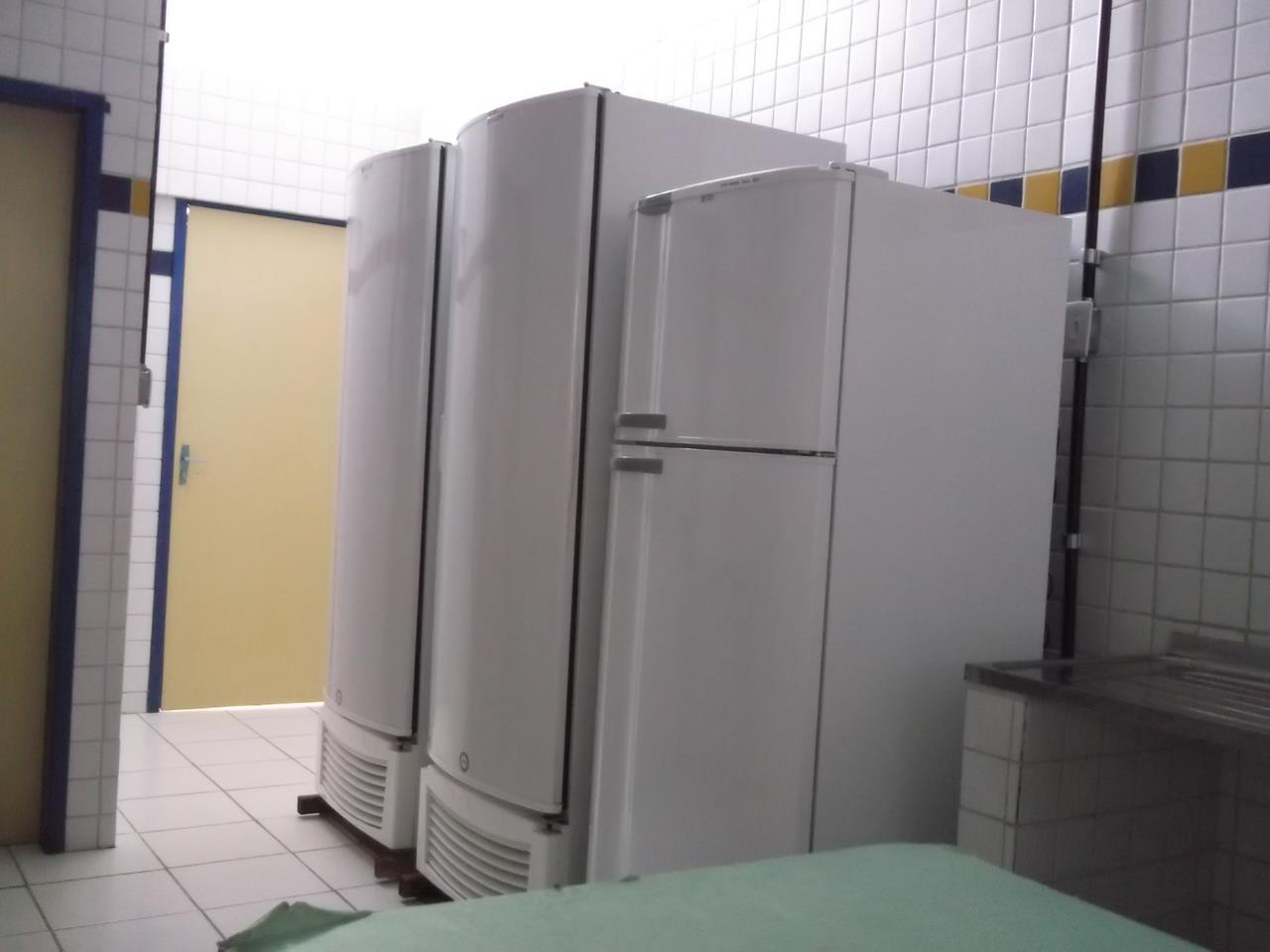The image depicts an industrial kitchen with walls adorned with small white tiles, interrupted by a horizontal line of yellow and dark blue tiles. The floor is covered with larger white tiles made of a different material. There are two beige doors with dark blue trims visible; one stands prominently in the background, while the other is partially seen to the left. The kitchen houses three white, shiny refrigerated units aligned in a row. The unit closest to the viewer features a freezer on top, while the other two units next to it appear to be large freezers with a single compartment. In the foreground, a table draped with a light green tablecloth is visible. To the left of this table, there is a dark-colored bench partially in view. The room has significant shadow, suggesting dim lighting, except near the background door, where the light is brighter.